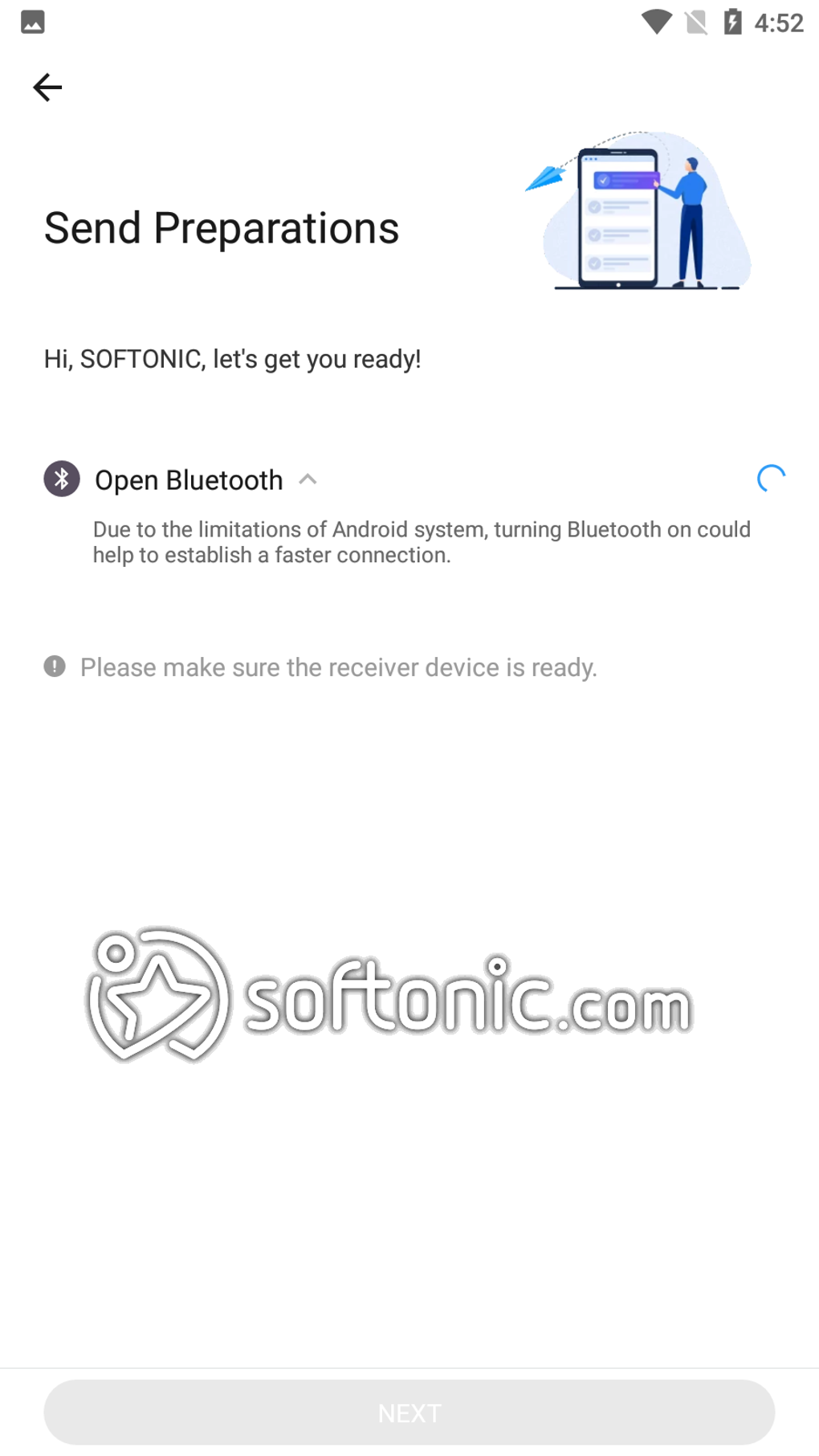### Detailed Caption:
In this image, we see a phone interface displayed in landscape mode, showcasing a setup guide by Softonic.com. The phone screen is devoid of SIM cards and shows no signal, but it is fully charged. The current time displayed is either 4:52 AM or PM. Wi-Fi is enabled, as indicated by the icon.

The header features a black back button on a white background. The centerpiece of the screen is an instructional message framed by a whimsical illustration: a man stands beside an oversized phone, tossing a paper airplane over it. The screen reads, "Hi Softonic, let's get you ready. Open Bluetooth." It further explains that enabling Bluetooth might expedite the connection due to Android system constraints, accompanied by a loading circle.

Below the instructions, there is a reminder to ready the receiver device. A small star within a circle hovers near the informative text. At the bottom of the screen, there's a faint watermark that reads "Softonic.com."

In the upper right corner, the illustrated man, dressed in dark blue jeans and a light blue work shirt, has thick, darker blue hair. He is interacting with the oversized phone, pressing a button that is now highlighted in purple. 

A grayed-out 'Next' button is also visible, awaiting activation to proceed. This setup appears to be part of Softonic.com's guide to initializing a new phone.